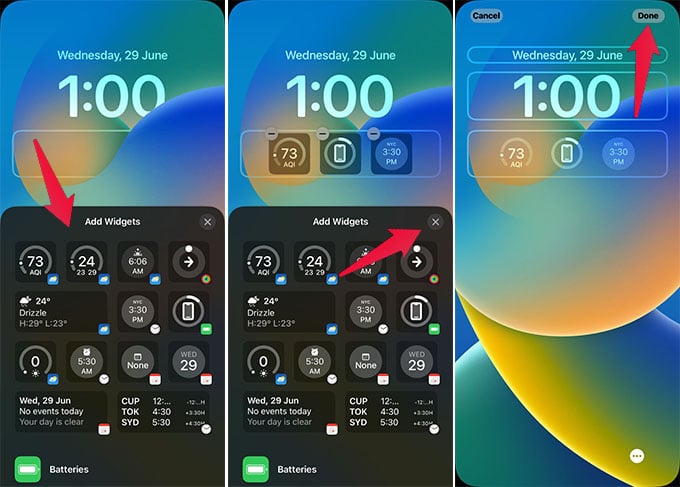**Detailed Caption for the Image:**

The image consists of three consecutive screenshots displayed side by side, illustrating a step-by-step guide on adding widgets to a smartphone's homepage. 

- **Screenshot One**: The interface shows the 'Add Widgets' feature in action, with a large red arrow pointing to the widget selection area where various widget sizes are available. The background reveals the smartphone’s homepage displaying the current date and time at the top.
  
- **Screenshot Two**: This view proceeds to show the homepage with three widgets successfully added underneath the date and time. A red arrow highlights the 'X' button next to the 'Add Widgets' option, indicating how to exit the widget selection menu.

- **Screenshot Three**: The final screenshot directs attention to the 'Done' button located at the top right corner via a red arrow. This screen confirms the completion of the widget arrangement process by instructing the user to finalize their changes.

Thus, these images comprehensively guide users through the process of adding, configuring, and finalizing widgets on their smartphone's homepage.